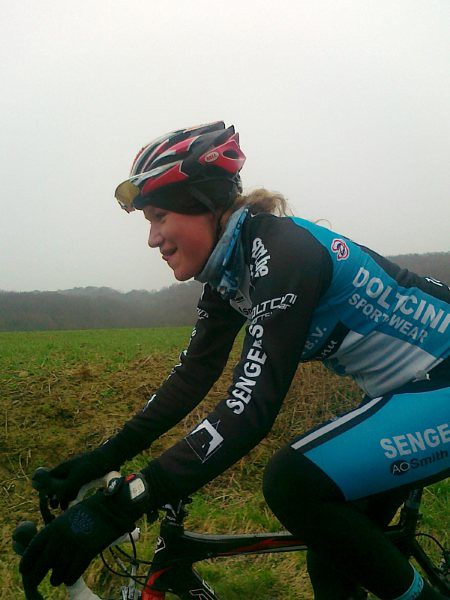In this image, a professional female cyclist is depicted riding her bicycle against a backdrop of green fields, rolling hills, and a gray, overcast sky. She is a Caucasian woman with a ruddy complexion, and she is smiling with her tongue out. Her helmet, which is red, black, and white, has a smooth, wavy design and sports white-framed sunglasses sticking out of it. The helmet partially reveals her blondish hair and covers some headgear underneath, likely for warmth. She wears a teal, black, and white cycling outfit adorned with various sponsorship logos, along with black gloves and a blue scarf around her neck. Additionally, she has a digital watch on her left hand. Her bicycle, mostly black with some red highlights, features partially visible logos in white.